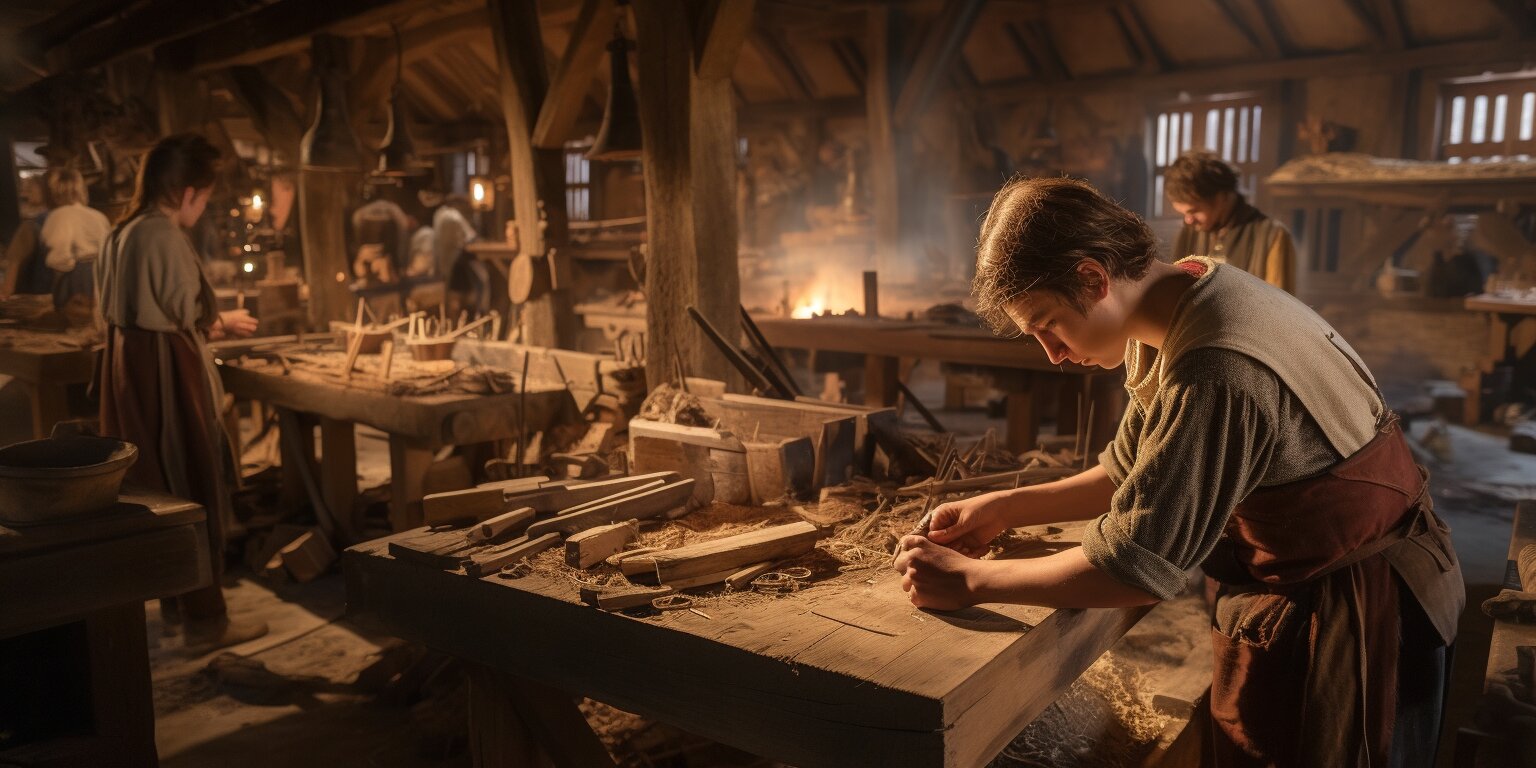The image, which could be a detailed painting, photograph, or even a computer-generated image, depicts an old workshop reminiscent of a renaissance-era or perhaps a 17th to 19th-century woodworking space. The scene takes place in what looks like an ancient, rustic room, possibly inside a barn, with wooden or stone walls and exposed rafters. A number of tables are scattered throughout, each occupied by individuals engrossed in woodworking activities. The foreground features a young boy with brown hair, dressed in an elbow-length top, long pants, and a brown sash, working diligently at a table laden with tools and wood shavings. To his left, a girl in similar muted clothing is carefully crafting another wooden object. At the back of the room, a fire burns in a fireplace, likely used for metalworking, contributing to the warm glow of the space. Several windows against the back wall allow light to filter in, illuminating the scene. The men and women, possibly young adults or teenagers, wear long, gray blouses with red aprons tied around their waists, embodying a historical aesthetic. The detailed features and the palpable sense of activity suggest a lively, bygone era workshop where skilled hands bring wood to life.